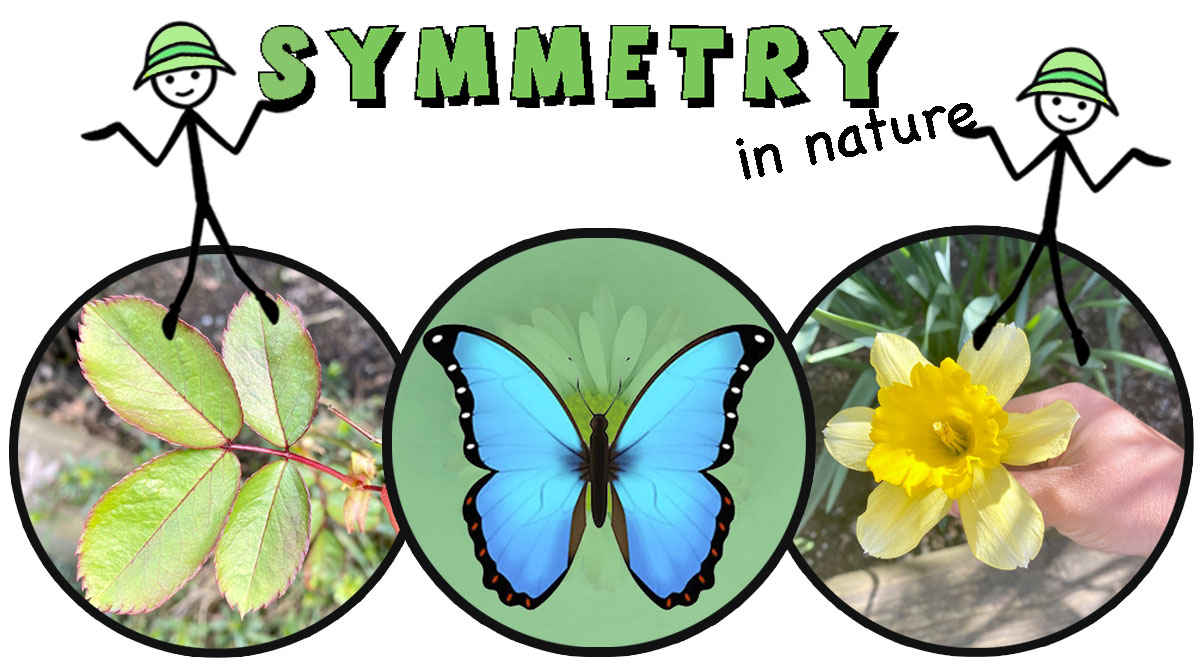This colorful illustration, reminiscent of a children's nature book or elementary science textbook, features a trio of overlapping circles, each depicting detailed elements of nature. The left circle showcases a close-up of green and red leaves, exhibiting intricate vein patterns. Central to the graphic is a blue butterfly with black-edged wings adorned with white and red dots, set against a green background with a hint of a small green flower. The right circle displays a vivid yellow daffodil held delicately by a human hand, the fingers partially visible around the flower. Above these images, the phrase "Symmetry in Nature" is prominently written, "Symmetry" in bold green and "in Nature" in black. Flanking this text, two whimsical stick figures in green gardening hats appear, emphasizing the theme of symmetry. This engaging and educational collage captures the harmonious patterns found in the natural world, making it an appealing illustration for young readers.